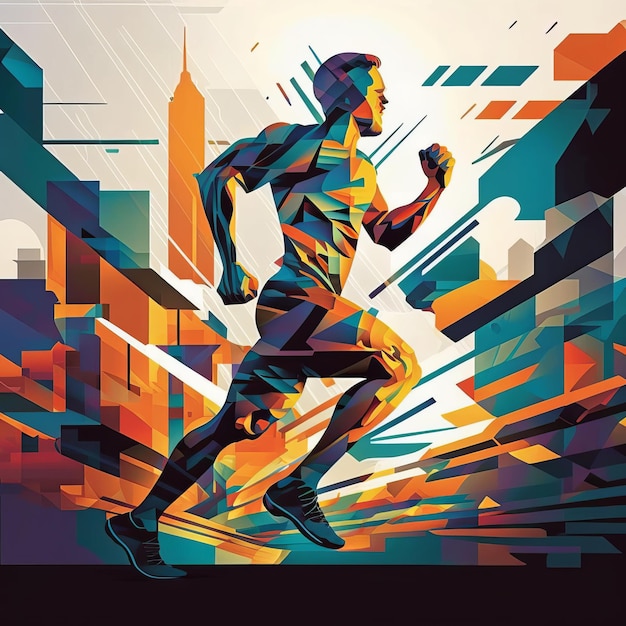This is an abstract digital artwork depicting the profile of a man running from left to right. The scene is rich with geometric shapes and vivid colors; the man himself is constructed from a blend of blues, golds, burnt oranges, and whites, with highlights of teal and purple. His form suggests dynamic motion, with one arm stretched forward and the other back, one foot planted on the ground, and the other raised mid-stride. He is wearing athletic shoes, although other fine details of his attire are obscured by the abstract design. The background is an explosion of color featuring a mix of orange, red, teal, and green tones, hinting at a cityscape. Notably, there is a shape that resembles the Empire State Building, adding to the urban aesthetic. The bottom border of the image is a solid black rectangle, grounding the vibrant composition.